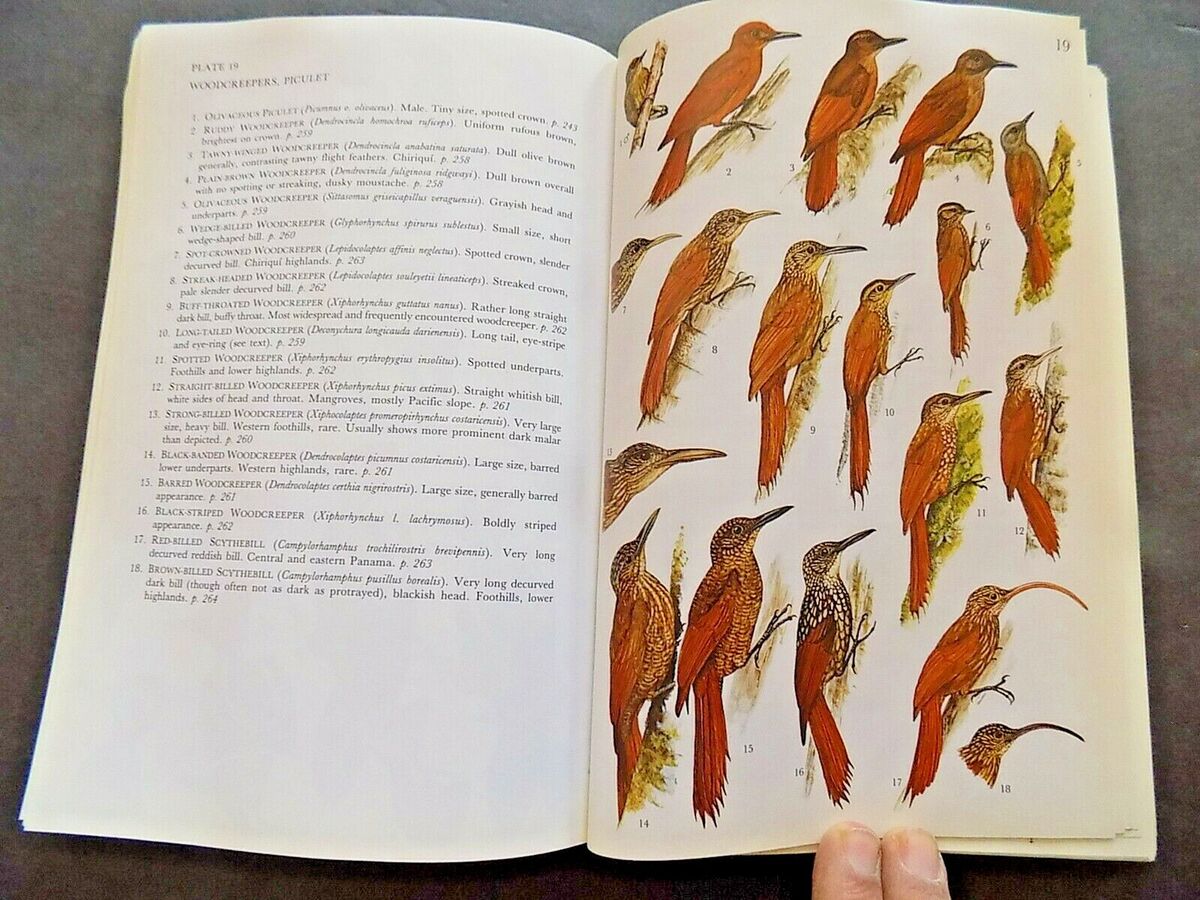This photograph captures an individual holding open an old book, the edges yellowed with age. On the left-hand page, titled "Plate 19," there’s a detailed catalog of woodcreepers, each identified with a common name, scientific name, and a description, such as the "Black-striped Woodcreeper," noted for its "boldly striped appearance," followed by a reference to "page 262." The list enumerates 18 different species, including "Brown-billed Side-bill" at number 18 and "Red-billed Side-bill" at number 17. The right-hand page features colorful illustrations of these birds, displaying variations in beak shapes and lengths, with many species sporting predominantly orange and reddish feathers. The drawings are meticulously detailed, showcasing birds with features like long, curved beaks. At the bottom of the right page, two fingers, presumably from the right hand of the person holding the book, are visible, gently touching the page to keep the book open.